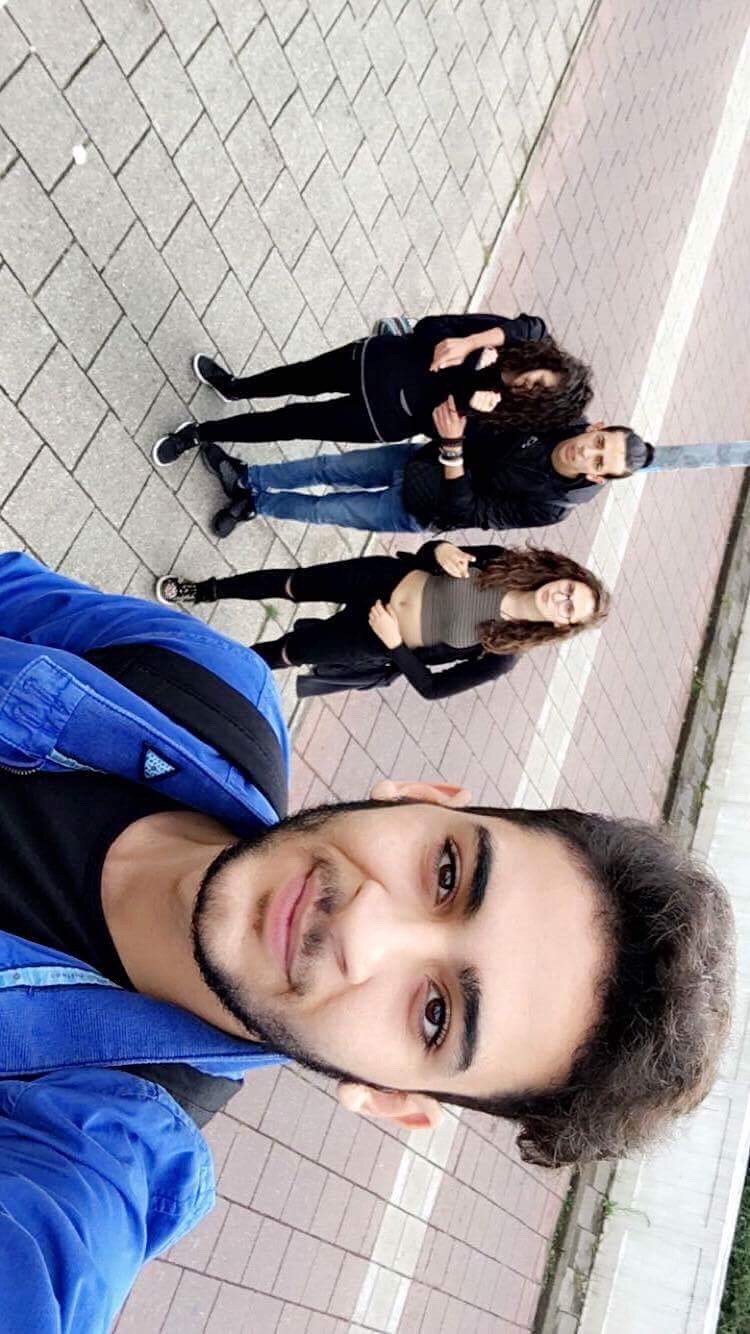This photograph, taken in color and turned on its side, captures a vibrant outdoor daytime scene featuring four young adults on what appears to be a paved sidewalk with distinctive brick and gray pavers. In the foreground, a young man with East Asian features, thick eyebrows, and a kind smile takes a selfie. He is wearing a bright blue jacket adorned with a black and white triangle on the collar, and a black t-shirt. His short brown hair is slightly poofy, and he sports a faint mustache and goatee.

Behind him to the upper-left, three friends pose together. The central figure, a man with dark hair pulled into a bun, wears blue jeans and a dark jacket. He has his arms wrapped around the shoulders of a girl to his left and another to his right. The girl on his left, partially hidden by her long wavy hair and hoodie, has her hands close to her chest. The girl on the right, distinguishable by her glasses, wears a gray crop top with black stripes, revealing her midriff, and black jeans with rips at the knees. She also playfully flashes a peace sign towards the camera. The overall scene is bright with no text visible in the image, capturing a candid and joyful moment shared among friends.